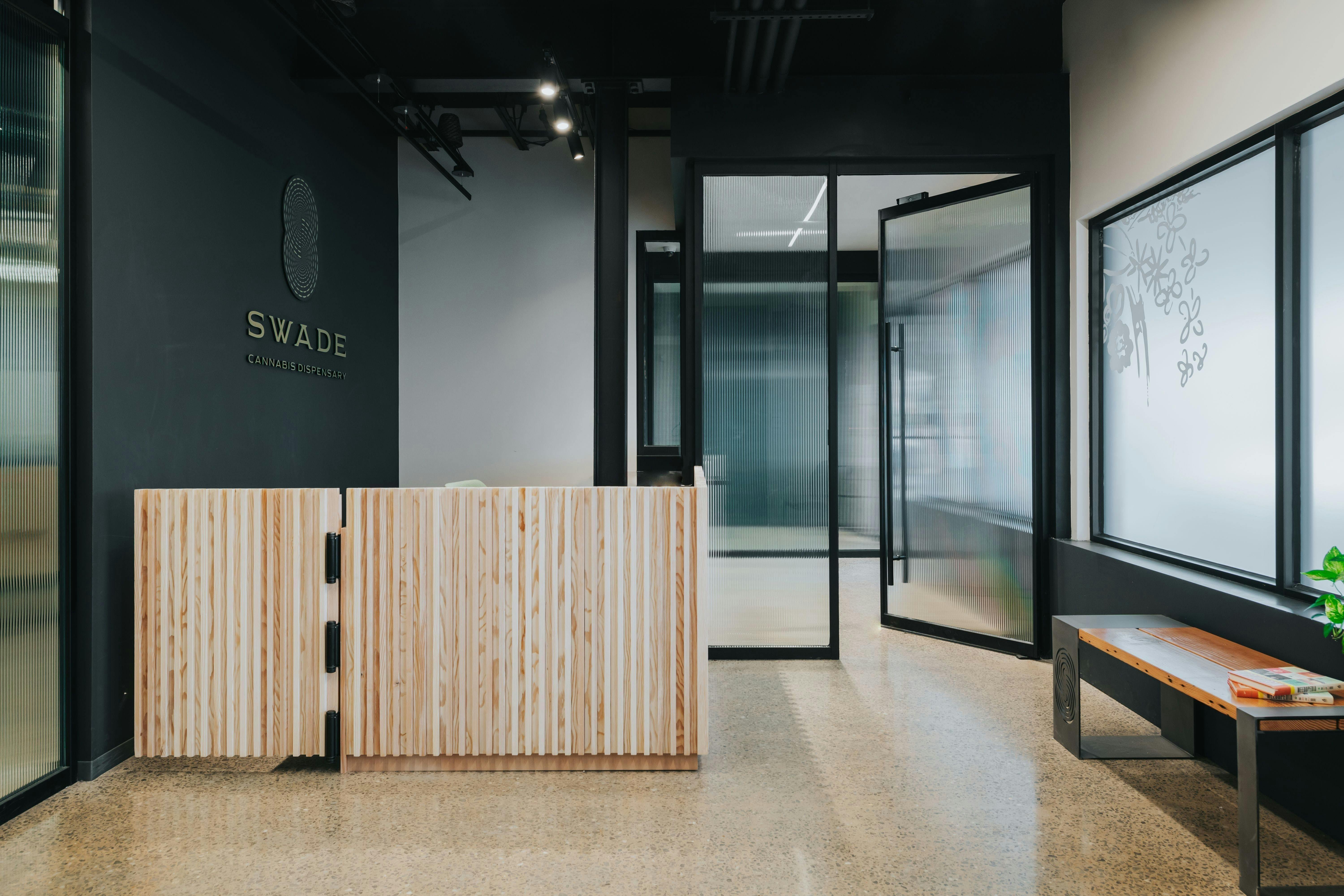The photograph depicts the lobby or reception desk area of an office building that exudes a highly professional and clean aesthetic. The lobby features floors with a combination of brown, cream, and tan tiles, complementing the charcoal-colored walls. Central to the lobby is a reception desk constructed from light-colored wood slats, situated below a corporate logo. The logo is a stylized letter "S" in a swirly gray pattern, with the name "Swade" (S-W-A-D-E) in gold letters beneath it. 

To the right of the reception desk, a window frames a black metal and wood bench, upon which rest two books. The entrance to this space is marked by a clear glass door with a black frame and a long black handle, which seems to lead into another smaller room that remains out of view. This immaculate setting suggests the building houses a company, possibly a legal firm or another business requiring a polished, professional atmosphere.